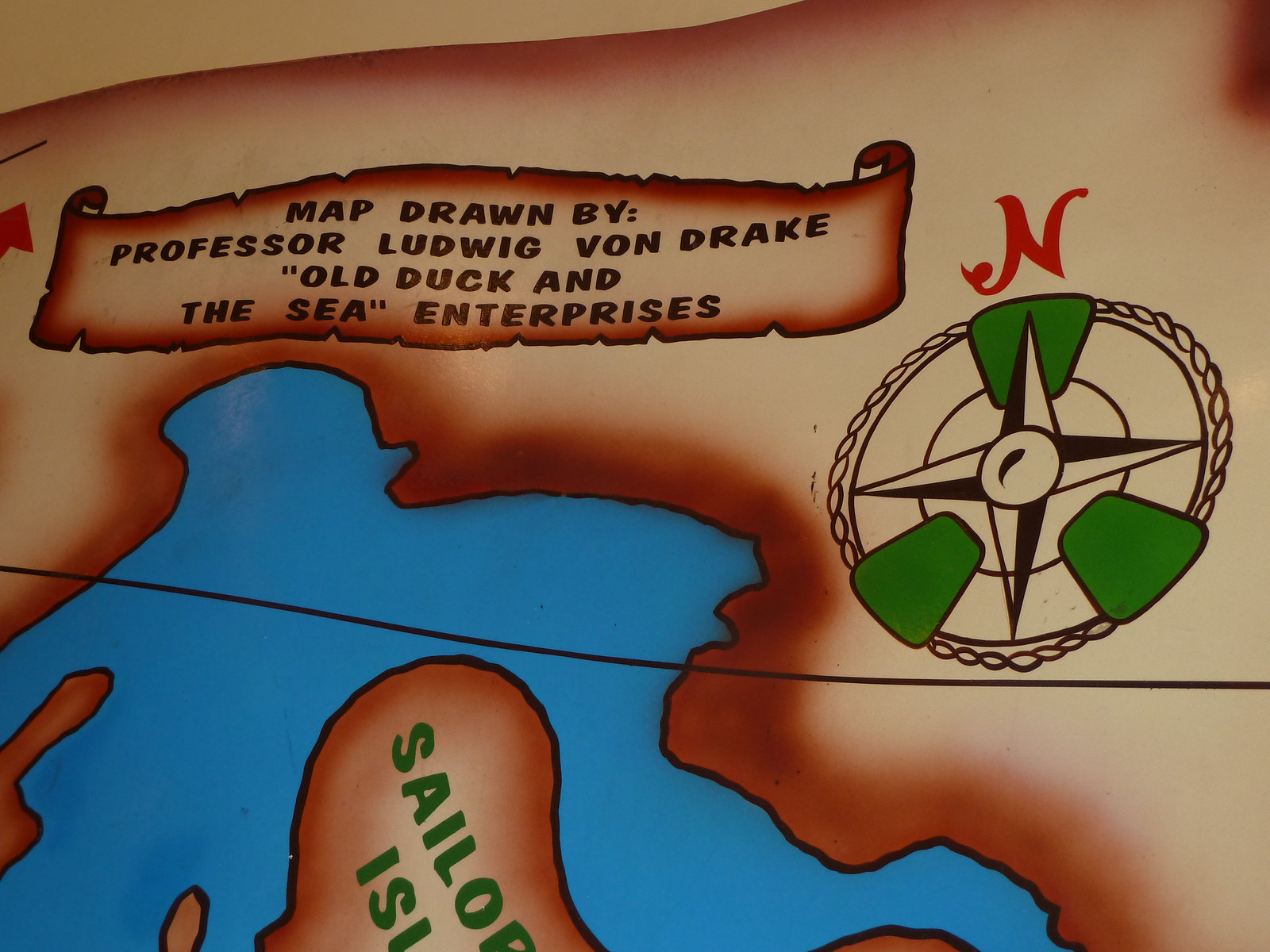This whimsical, hand-painted map exudes a playful and childlike charm. Dominated by vibrant hues of green, red, brown, and blue, it features a quirky depiction of an island named "Sailor Island," although the full name is partially obscured. Nestled among a wash of surrounding waters, the island is intricately illustrated to captivate the viewer's imagination. A compass rose, skillfully drawn in the top right corner, indicates north as being upwards, adding to the traditional map elements. Near the top of the image, a strip of parchment - painted with dark brown text - reads "Map drawn by Professor Ludwig von Drake, Old Duck and the Sea Enterprises," lending a humorous and narrative touch. The image is closely cropped, offering a tantalizing glimpse into this delightful and meticulously crafted cartographic creation.